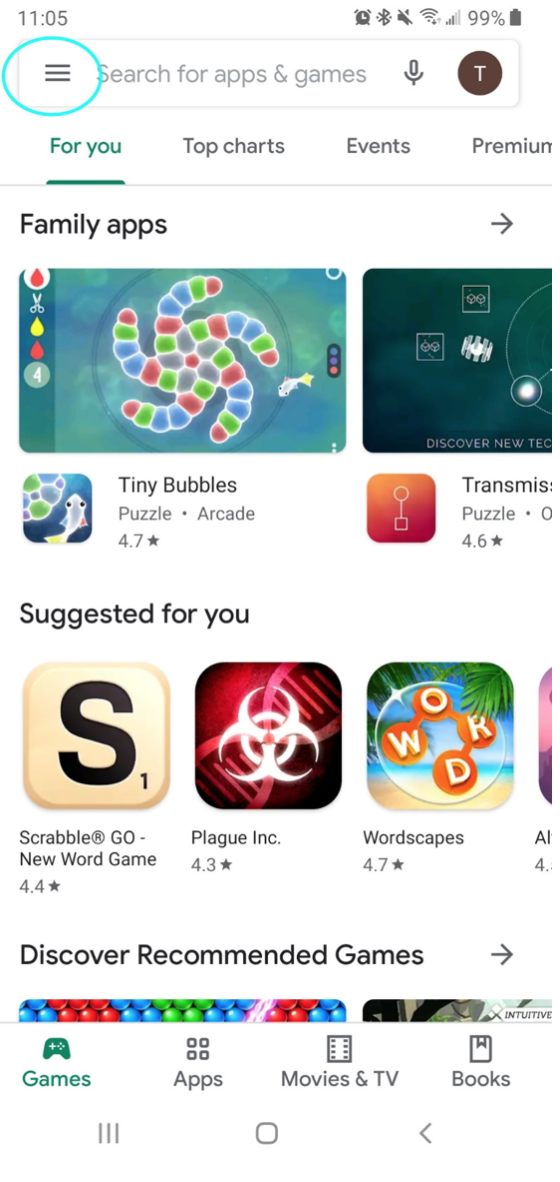The screenshot, taken on an Android device, displays the Google Play Store interface. The time on the device is 11:05, and it shows multiple status icons: alarms set, Bluetooth enabled, phone on silent mode, a Wi-Fi signal at three out of five bars, and a battery level at 99%.

The main focus of the screenshot is a pale blue circle highlighting the "hamburger" menu icon, consisting of three horizontal lines stacked on top of each other, commonly used to access a menu. Directly above this icon is a search bar that says "Search for apps & games," which includes options for both text input and voice search, indicated by a microphone icon.

Displayed prominently below the search bar is a section titled "For You," highlighted in blue with a blue underline. Other visible tabs include "Top Charts," "Events," and "Premium." Underneath these tabs, there's a horizontal list labeled "Family apps," with a right-pointing arrow, suggesting more content can be viewed.

A highlighted portion features the app "Tiny Bubbles" in the "Puzzle & Arcade" category, boasting a rating of 4.7 stars. Partially visible apps include a puzzle game with a 4.6-star rating and "Scrabble GO," marked with a Scrabble tile icon and a 4.4-star rating. Other apps displayed in the "Suggested for You" section are "Plague Inc." with a 4.3-star rating, "Wordscapes" with a 4.7-star rating, and another cut-off app icon.

At the bottom of the highlighted area, there are various sections like "Games" indicated by a game controller icon, "Apps" shown with four little squares, "Movies & TV" represented by a film reel, and "Books" marked by a book icon with a bookmark.

Overall, the screenshot highlights a comprehensive and user-interactive layout within the Google Play Store app, detailing various options for browsing and discovering new apps and games.